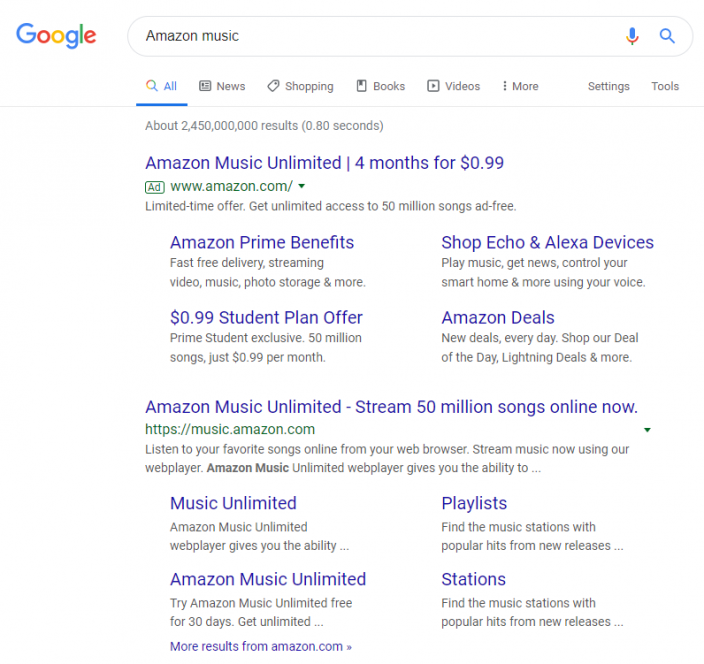The image shows the Google search results page for the query "Amazon Music." At the top, the familiar search bar is visible, complete with the microphone and magnifying glass icons on the right. The search query is already typed in. The navigation tabs below the search bar display options such as "All," "Shopping," "Books," "Videos," "More," "Settings," and "Tools," with the "All" tab highlighted in blue and underlined. 

The search results indicate a total of approximately 2,450,000,000 results retrieved in 0.8 seconds. The top result is a clearly marked ad for Amazon Music Unlimited, offering a promotional rate of four months for $0.99. The ad is from amazon.com and promises access to 50 million songs, ad-free, as a limited-time offer. 

Beneath the top ad, there is a two-by-two grid featuring four promotional links: "Amazon Prime Benefits" to the top left, "Shop Echo and Alexa devices" to the top right, "$0.99 student plan offer" on the bottom left, and "Amazon Deals" at the bottom right. 

Following this grid, another link for Amazon Music Unlimited appears. It directs users to music.amazon.com, boasting the ability to stream 50 million songs online. This link is accompanied by four further inset options: "Music Unlimited," "Playlists," "Amazon Music Unlimited," and "Stations," each with a brief description.

At the bottom of the search results, there is a link for more results from amazon.com, ensuring that users can easily find various Amazon Music-related information. 

The overall atmosphere of the search results emphasizes the ease of finding and accessing Amazon Music through Google.